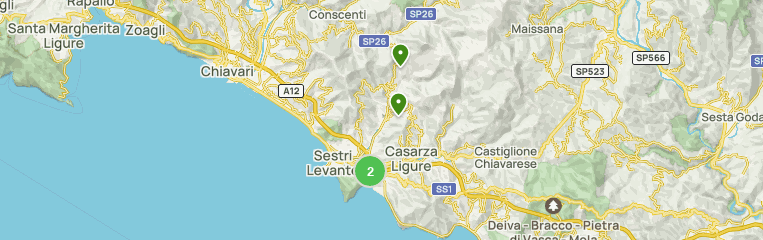This image showcases a computer-generated map, primarily featuring a region near a body of water on the left side, which occupies a little under half of the photo in shades of blue. The map itself is horizontally rectangular and depicts the land in soft light gray tones, with roads highlighted in yellow. Several towns and cities are labeled in black letters, such as Santa Margarita, Liguerre, Zoagli, Chiavari, Consente, Cestra, Levante, Casarga, Castiglione, Chiaveres, Delba, Braca, and Pietra. Notably, a green circle with the number two highlights Sestri Levante. The presence of labels like SP-26, SP-23, and SP-566 suggests a structured road system. The map's place names hint at a region influenced by Hispanic or Italian linguistics, as illustrated by the spellings and pronunciations of the locations.